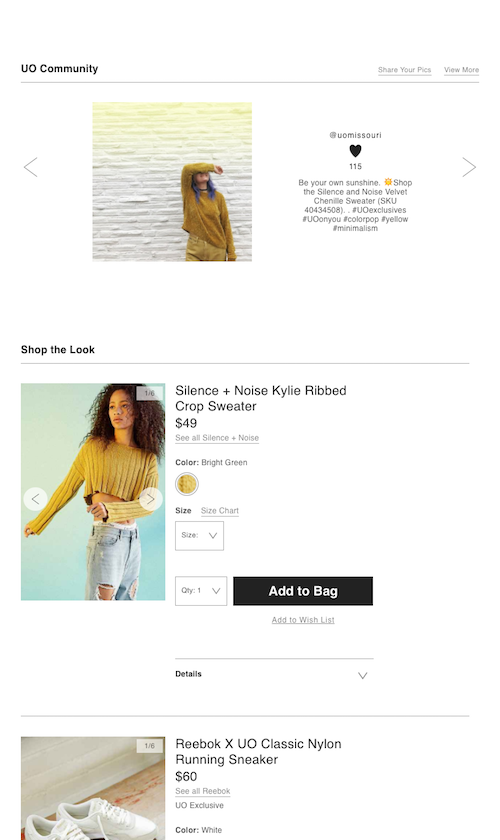**Caption:**

The webpage titled "UO Community" features buttons at the top for users to share their photos or view more content. The first post showcases a user with the handle **@UOMissouri**. It has received 115 likes, indicated by a black heart icon, and bears the caption: "Be your own sunshine ☀️. Stop the silence and noise. Velvet phenyl sweater SKU: 40434508." Accompanying this post is a photograph of a person wearing a vibrant yellow sweater, with their hand shielding their eyes. The individual, who has purple hair, stands against a backdrop of a white and yellow brick wall. The post includes hashtags: #UOExclusives, #UOonU, #ColorPop, #Yellow, and #Minimalism.

Just below, another image invites users to "Shop Your Look." The description reads: "Silence, Pleasant Noise. Kylie Ribbed Crop Sweater - $49." The sweater is a bright green color, modeled by a person wearing distressed jeans. Options are available for selecting a size, displayed alongside a size chart and a prominent black "Add to Bag" button.

The final listing highlights a "Reebok x UO Classic Nylon Running Sneaker" priced at $60. The section encourages viewers to "See All Reebok UO Exclusive." The sneakers are traditional white with laces, perfectly captured in the accompanying image.